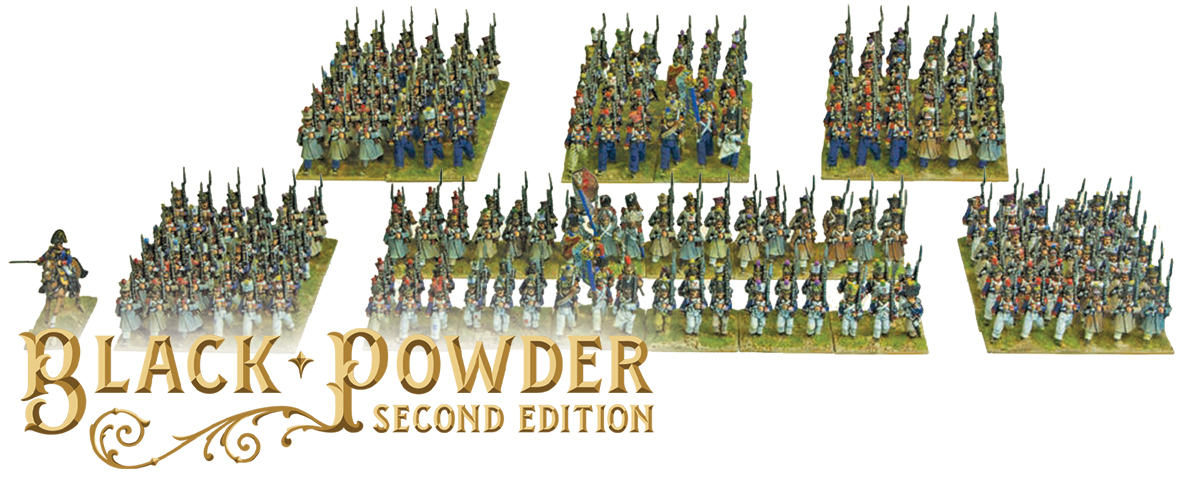The image depicts a collection of miniature toy soldiers, associated with the game "Black Powder, Second Edition." The gold Gothic-style text "Black Powder, Second Edition" is prominently displayed at the bottom. The figures are arranged on square or rectangular patches of green terrain, simulating battlefield formations. There are six distinct clusters of soldiers: three in the background composed of nine rows of five figurines, and three in the foreground with two squares on the ends and a larger rectangular section in the center. The soldiers are detailed with varying uniforms, predominantly in shades of blue, indicating different ranks or units. Some uniforms are dark blue, while others are light blue, and most soldiers wear hats. Among the figures, there is a notable soldier on horseback, distinguished by a fancy military hat and a sword. Additional soldiers appear armed with rifles, some equipped with bayonets. The total count of figurines is estimated to be between 50 and 60, all positioned against a white background.